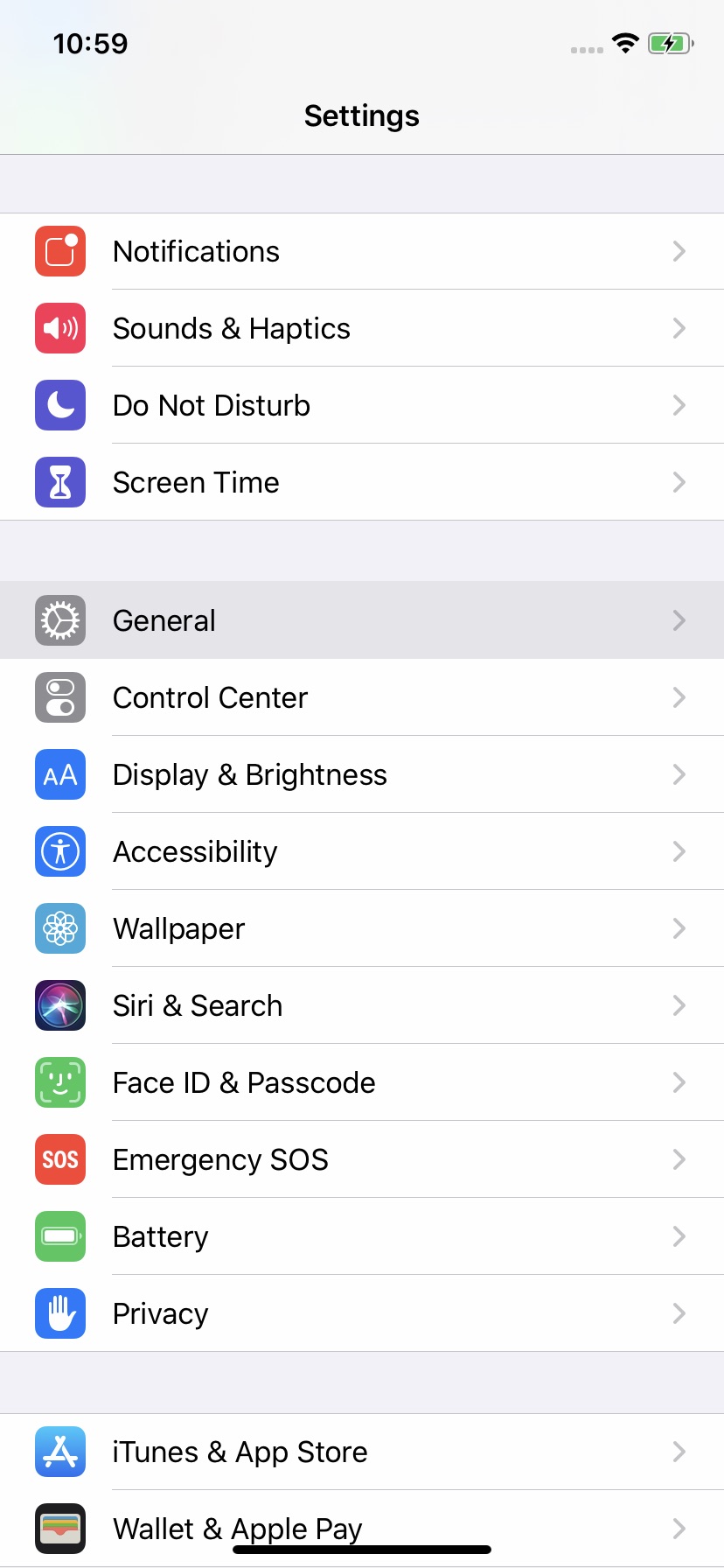This image appears to be a screenshot from a smartphone displaying the "Settings" menu. At the very top, there's a light gray status bar. In the upper left corner, the time is shown as 10:59, and to the right, the status icons indicate active Wi-Fi and an almost full battery. Centered at the top, the title "Settings" is displayed.

Below the title, there are four main settings categories, each with an icon:
1. **Notifications**: Represented by a red square with a white square and dot inside.
2. **Sounds & Haptics**: Depicted with a red square containing a speaker emitting sound waves.
3. **Do Not Disturb**: Indicated with a moon icon.
4. **Screen Time**: Shown with an hourglass icon.

Following these, the next group of settings includes:
1. **General**: Accompanied by a gear icon.
2. **Control Center**: Featuring an icon with two buttons.
3. **Display & Brightness**: Marked with a blue square containing two small triangles.
4. **Accessibility**: Identified by a blue square with a figure inside a circle.
5. **Wallpaper**: Represented by a teal square with a white graphic resembling a flower.

Additional settings listed below these include: "Siri & Search," "Face ID & Passcode," "Emergency SOS," "Battery," and "Privacy." Finally, at the bottom, two more options are visible: "iTunes & App Store" and "Wallet & Apple Pay."